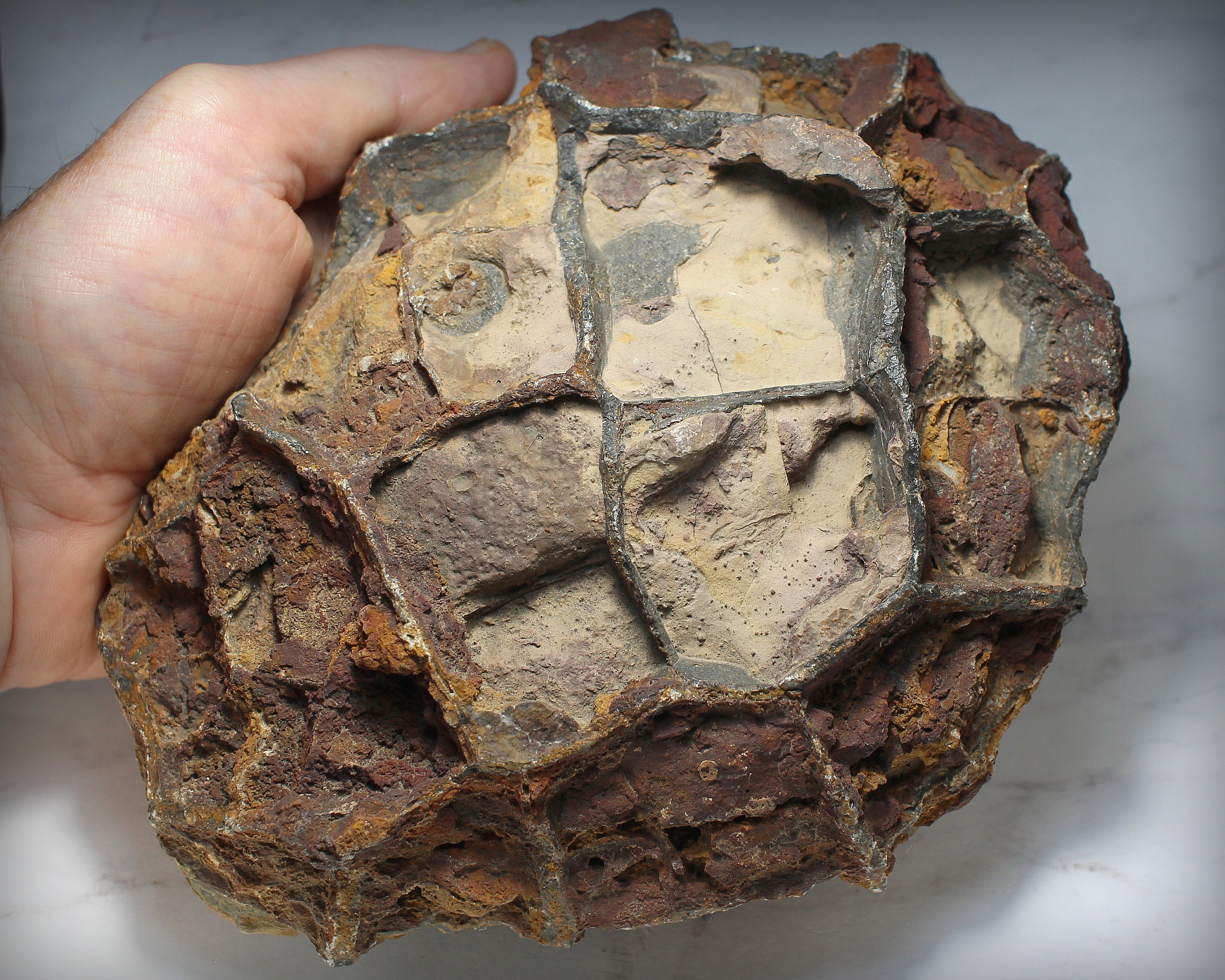The image is a square, full-color photograph taken indoors under artificial lighting, clearly staged, and featuring a plain but somewhat shadowy background in shades of white and light gray. The focal point of the image is a large, fossil-like, stone object being held in a Caucasian man's left hand, visible at the edge of the frame. The hand shows the thumb, part of the palm, and wrist, hinting at the object's considerable size that exceeds the width of the hand. The stone object appears weathered and features complex patterns and color variations, including browns, tans, grays, creams, and occasional touches of red and yellow. Its surface seems textured with crisscrossing lines and segmentations, reminiscent of a septarian nodule or fossil with potentially distinct boxed areas separated by darker gray lines, evoking a sense of geological and archaeological significance.